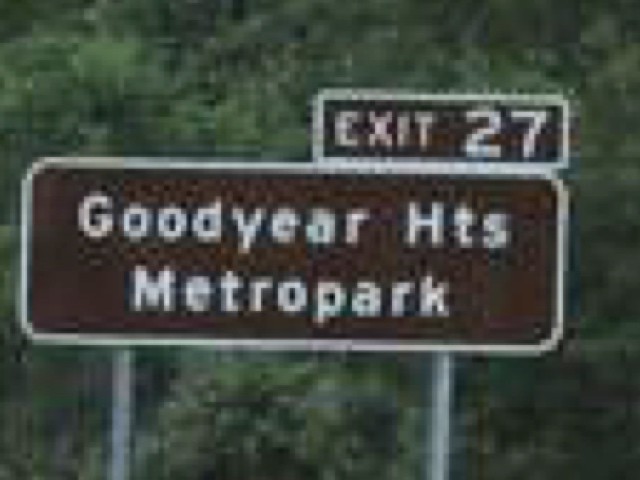This photograph depicts a somewhat blurry and pixelated image of a road sign against a backdrop of lush green trees, indicating that it was likely taken during the spring or summer. The main rectangular sign, horizontally oriented with rounded corners and stepped edges, is dark brown or burgundy with white text reading "Goodyear HTS Metro Park." Above it, on the top right corner, a smaller sign is attached, displaying "Exit 27" also in white text. Both signs are outlined in white and are mounted on two silver metal poles. The image's focal point, the road sign, is centered in the frame, standing out clearly against the indistinct, leafy background that suggests a forested area. Despite the significant pixelation and compression artifacts, the signage remains legible.